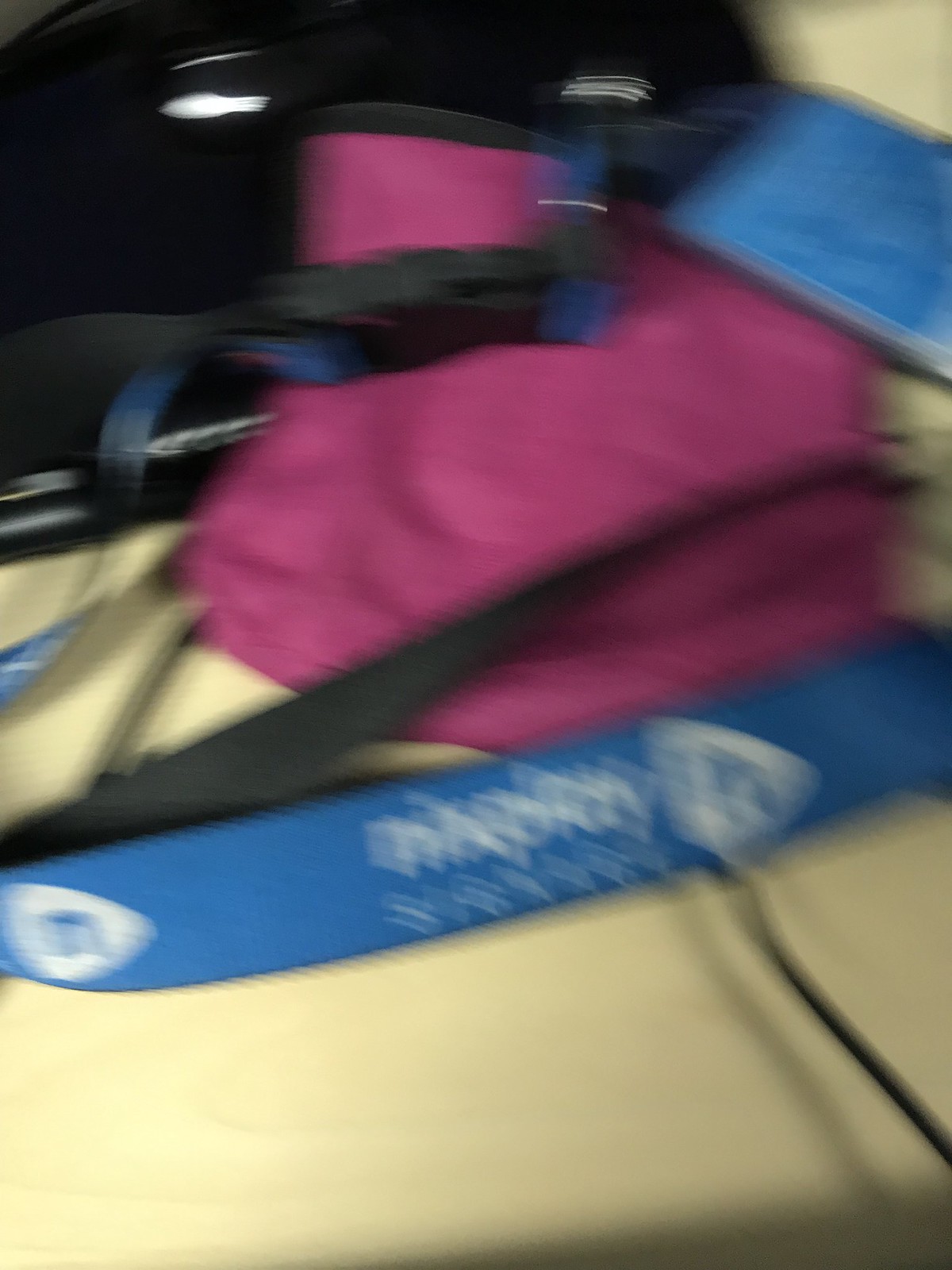This photograph captures an out-of-focus scene that appears to feature various items, dominated by a mixture of straps and cords. Among the elements is a black, indistinct object placed prominently in the foreground. Behind it, a series of black straps and buckles reminiscent of those found on a backpack are visible. Adding a touch of color to the composition is a mauve plum-colored sack, situated somewhat in the background and partially obscured by the straps. The lack of clarity in the image makes the exact nature of the objects challenging to discern.